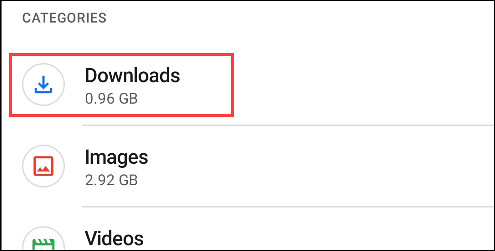The image captures a partial screenshot from a digital device, either a computer or smartphone, with a white background. Two faint horizontal gray lines are visible, adding minimal structure to the interface. In the upper left-hand corner, "CATEGORIES" is written in medium gray, capital letters. Directly beneath this, a red rectangular outline frames the word "Downloads" written in black text, accompanied by the data size "0.96 GB". To the left of "Downloads" is a blue download icon, featuring a downward-pointing arrow atop a horizontal line. Further down, in bold black text, the word "Images" appears, with the corresponding data size "2.92 GB" listed below. This section is marked by a small square icon representing images. At the very bottom of the visible area, the label "Videos" is partially obscured, with only the top portion of its green icon visible, and the data size for this category is not shown.